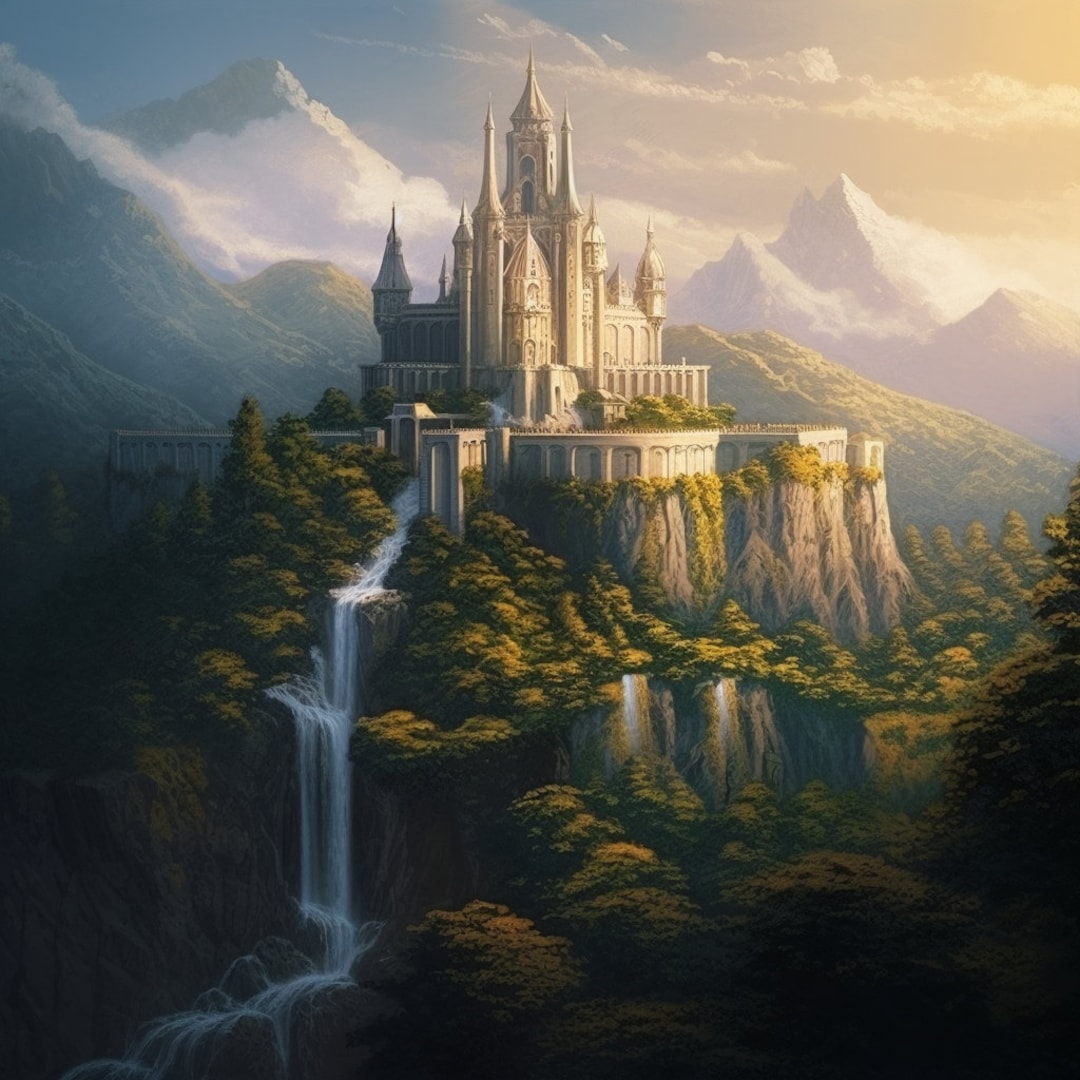The image depicts a highly detailed and stylized illustration, possibly a painting or computer-generated rendering, of an elaborate fantasy castle perched atop a hill. The extensive and ornate structure, which exudes a bright, cream or marble-like appearance, features numerous turrets and pillars. The hillside beneath the castle is lush with trees and includes cascading waterfalls that appear to emerge from the castle walls. Behind the castle, the scene reveals a sunlit sky with white-capped mountains and clouds, possibly indicating either sunrise or sunset. The background mountains display a mix of snow and greenery. The imagery is indicative of a scene from a video game, comic book, or virtual reality, characterized by vibrant colors, including dark tones, greens, yellows, grays, and whites. Notably, there is no text present in the image.